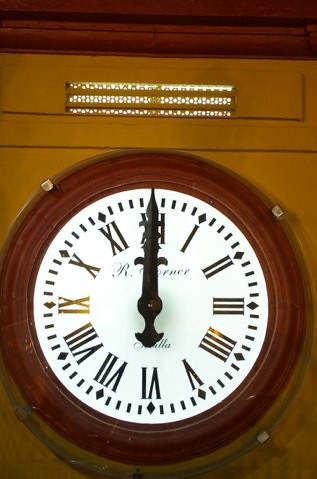The image features a large, vintage clock mounted on the interior wall of a building. Positioned directly below a ceiling vent, the clock is encased in a wooden frame, accented by four gold fasteners securing its facade. At the top of the wall, intricate wooden molding adds a touch of elegance to the setting. The clock is designed in an old-fashioned style, displaying the time as exactly 12 o’clock. Its face is adorned with Roman numerals, rendered in a gleaming metallic finish. The name of the clockmaker, partially obscured by the hour and minute hands, appears to be "R. Corner."